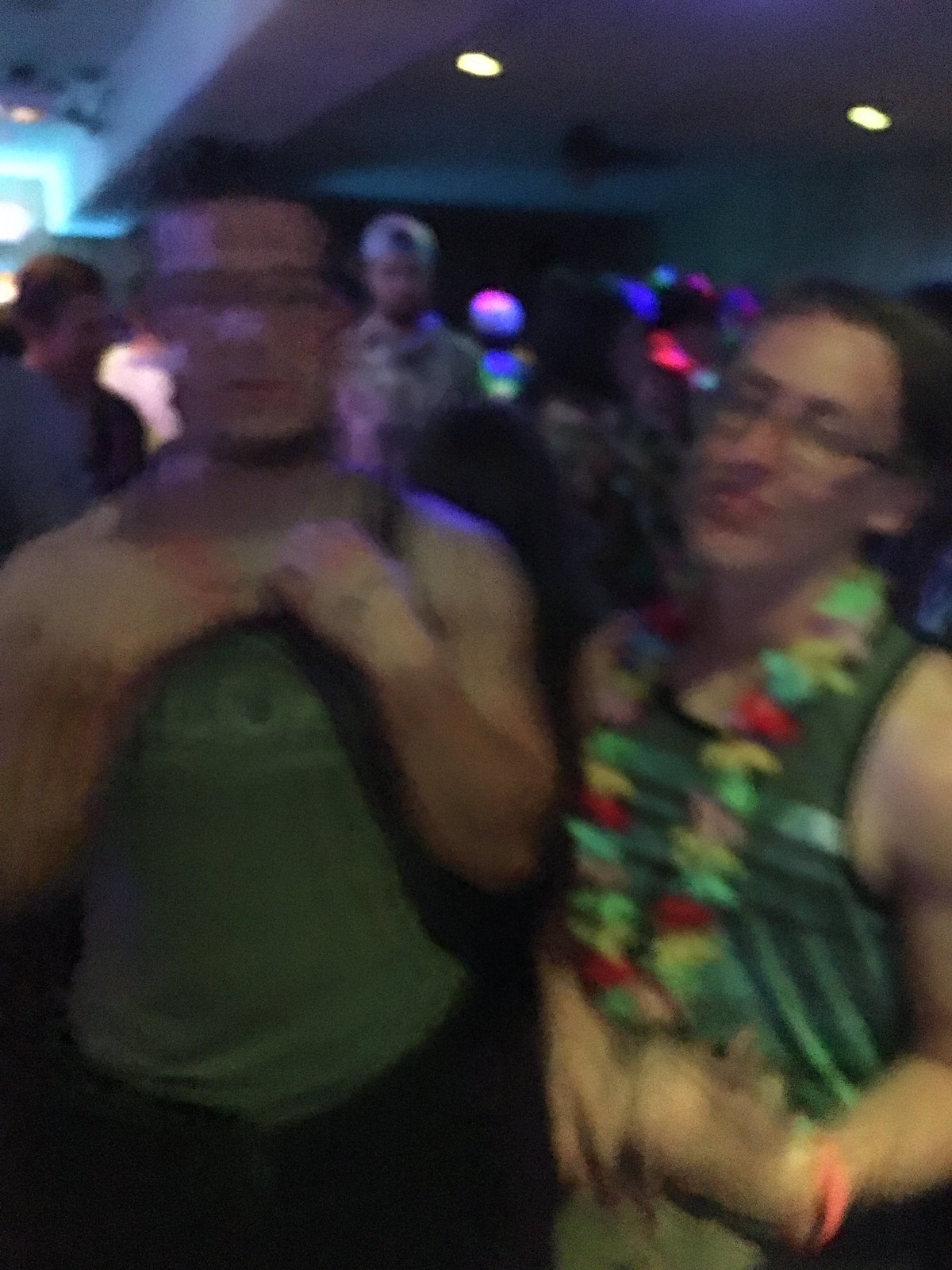The image captures an indoor scene, possibly inside a dimly lit club or party venue, characterized by its blurred and grainy quality. At the forefront, two individuals stand out prominently. On the right, a person, whose gender is ambiguous, sports short hair, glasses, a green tank top, and a multicolored Hawaiian lei with hues of green, red, yellow, and gray. They have a pinkish-orange bracelet on their right wrist and appear to have both arms bent with hands placed around their stomach area. On the left, another individual, presumed male, is wearing a greenish sporty tank top and glasses. His arms are bent at the elbows and positioned near his chest. He too has short dark hair and a distinctive black band around his neck, with possibly a stamped marking on his right arm. Both central figures seem to be facing the camera in an action shot, adding to the overall blurriness.

In the background, the dim environment continues with various people vaguely visible. Notably, there is a man with a patterned top and a backwards white baseball cap located a little left of center. Two space-style lighting fixtures are recessed into the white ceiling, providing minimal illumination along with some subtle light visible from the upper left corner. Additional blurred figures are seen to the left of the central man, contributing to the impression of a crowded and lively venue. Overall, the photograph’s details assemble a scene reminiscent of a night out at a bustling club or party.